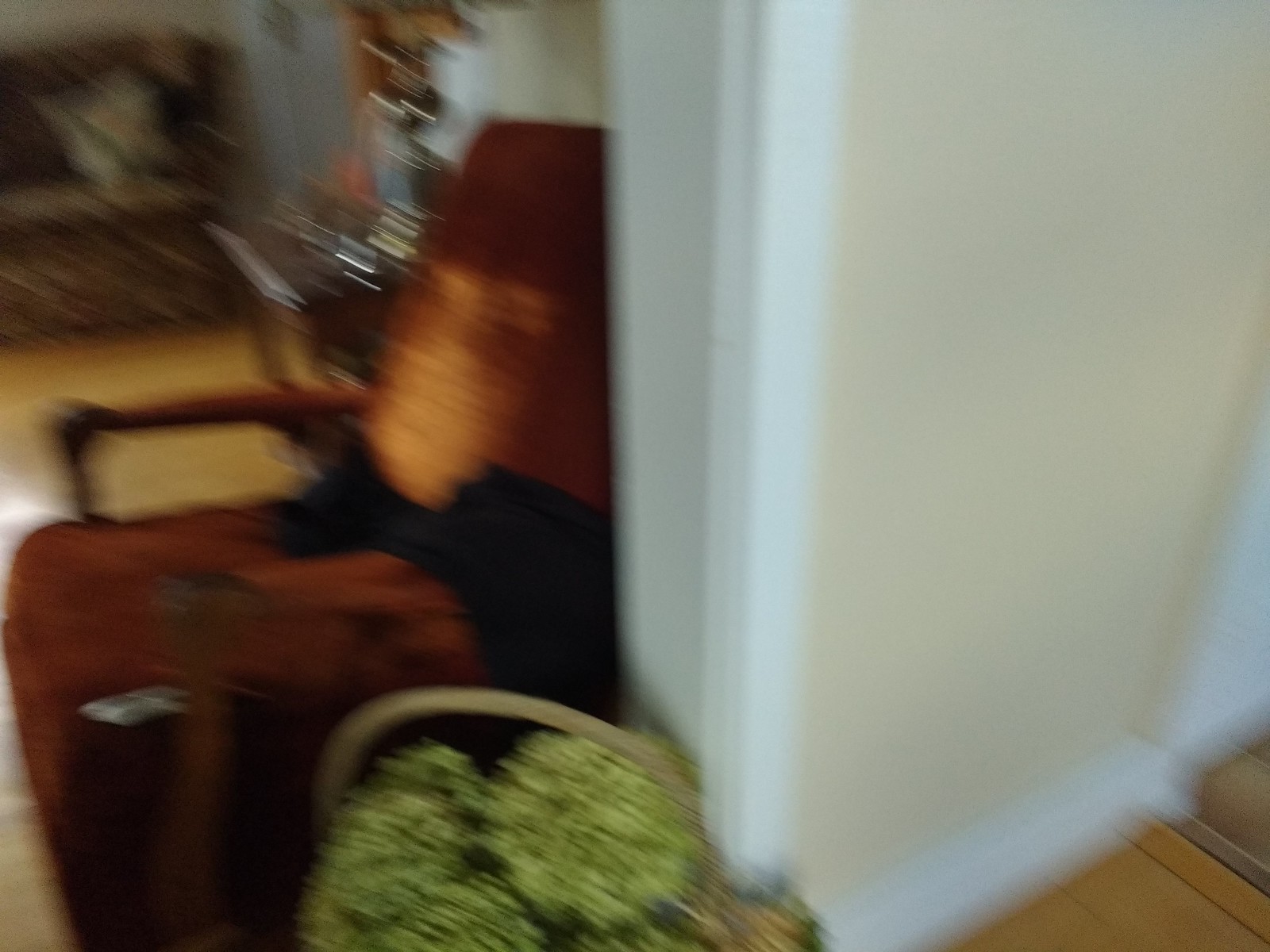This photograph, taken from a hallway looking into a living room within a house, is notably blurry but reveals a cozy, detailed interior. A light wood-stained floor leads up to a white-painted arched entryway, which frames the scene. Prominently positioned on the floor at the arch is a wicker basket with a handle, brimming with pale green and white flowers, giving it a full appearance. Just beyond this basket, a dark orange or rust-colored armchair sits, possibly made of velvet, distinguished by its dark wooden arms and adorned with a black cloth or throw blanket draped over its seat.

The living room extends behind the chair, with wooden flooring continuing throughout. Adjacent to the chair is a wall or column that separates the seating area from the rest of the space. A side table in dark wood, featuring stacked books and a lamp, stands nearby, complementing the cozy ambiance. In the background, a couch with a green, cream, and black patterned throw pillow is positioned to face the doorway. The overall scene, though blurry, conveys a sense of homely warmth and detailed organization.